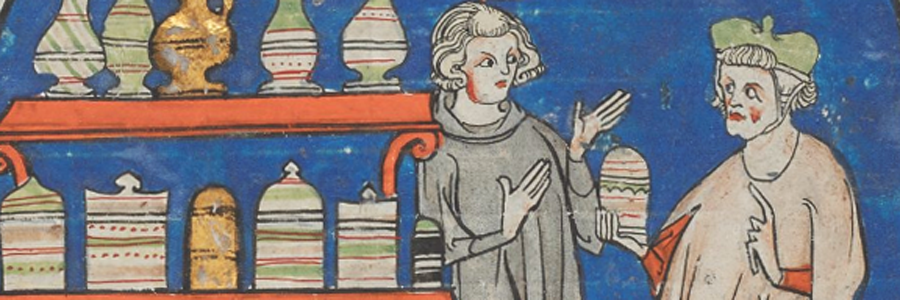This horizontally oriented hand-drawn artwork depicts a vibrant scene that appears to be set in the 1500s or 1600s. The background of the entire piece is a rich dark blue, accentuating the colorful elements in the foreground. On the left side, there is an orange shelving unit filled with various multi-colored ceramic pieces, ranging in shades from white and beige to green, pink, and yellow. The pottery is detailed, with some featuring horizontal stripes.

The central focus of the image is on the right, where two individuals are engaged in conversation, possibly negotiating over ceramics. Both characters are only visible from the waist up. The person on the left is dressed in light gray robes, has white hair, red lips, and their hands are outstretched as if discussing. The person on the right is clad in light pink robes with red sleeves and a green hat, holding one of the jars from the shelf in their right hand while pointing with their left, emphasizing their words.

The arrangement highlights the contrast between the structured display of ceramic goods on the left and the dynamic interaction between the two individuals on the right. The overall composition and detailed coloring bring the historical and commercial aspects of the scene to life.